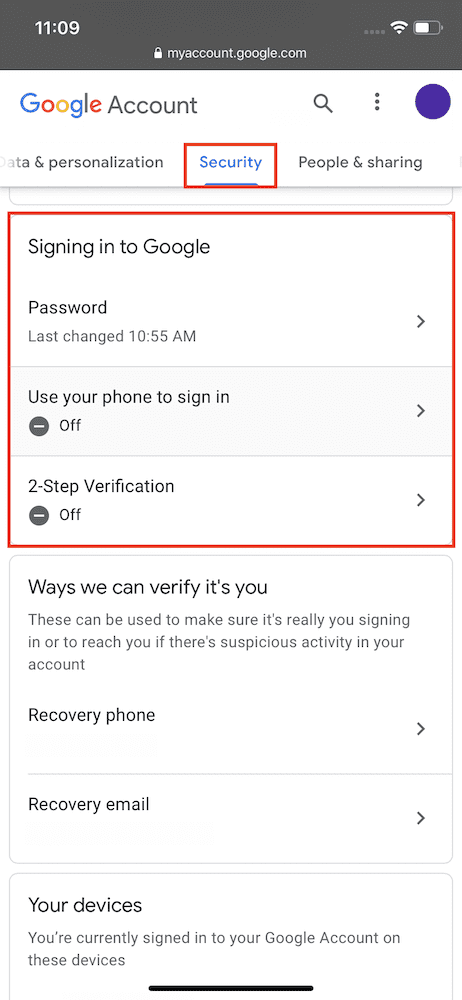A smartphone screen displays the 'myaccount.google.com' webpage, specifically open to the Google Account security page. Positioned at the top is the title, "Google Account", along with several tabs including 'People and Sharing' and 'Data and Personalization'. The 'Security' tab is currently selected. Beneath this, there is a section titled "Signing in to Google" showing that the password was last changed at 2:55 a.m. The page includes security features such as 'Use your phone to sign in' and '2-Step Verification'. Further down, there's a segment labeled "Ways we can verify it’s you," which offers options for 'Recovery phone' and 'Recovery email' to help verify your identity or contact you in the event of suspicious activity. At the bottom of the page, there's a section titled "Your devices," listing the devices currently signed into the Google account.